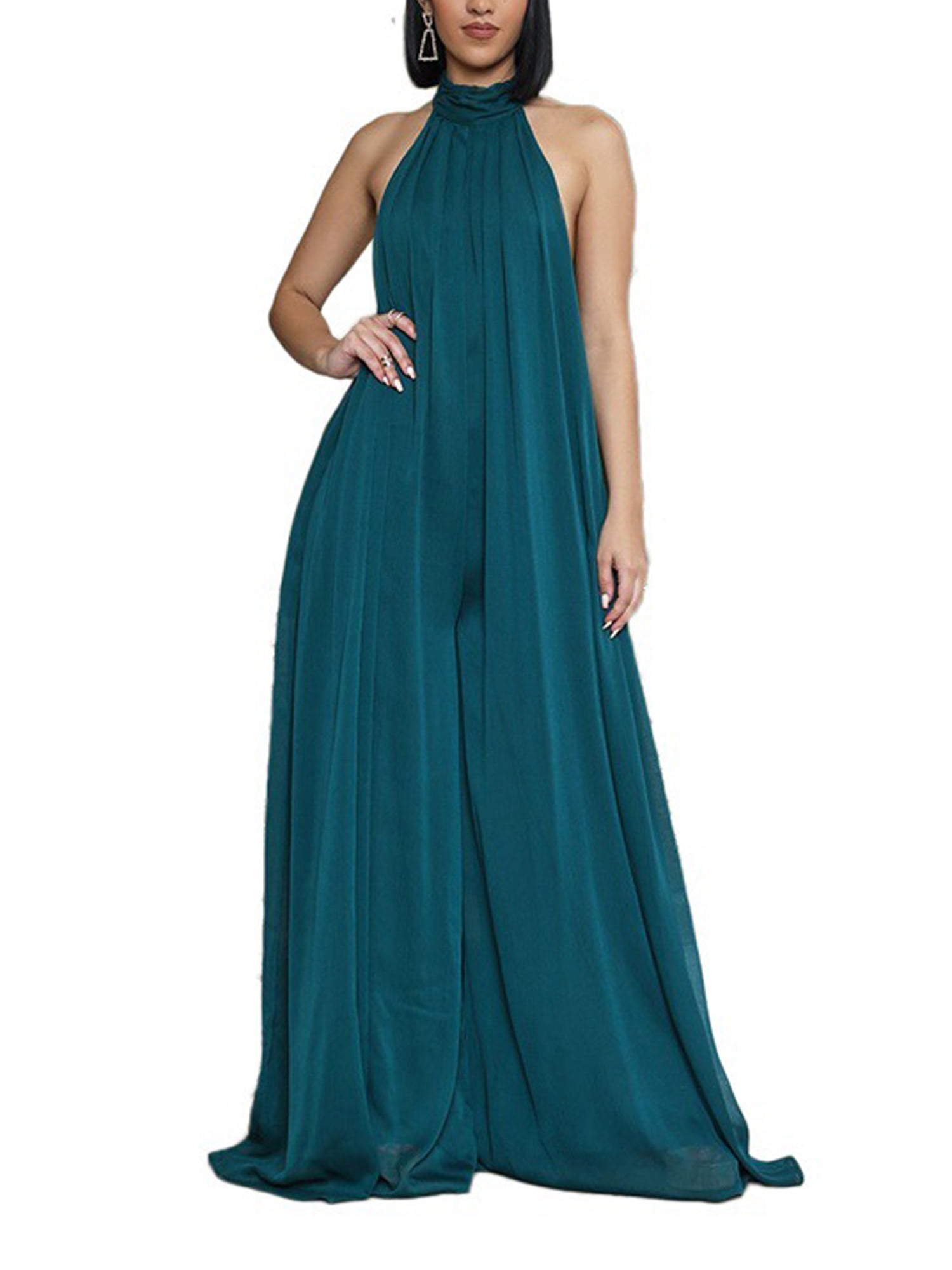The image is a photograph of a woman in a sleeveless, deep teal dress or gown that spans from the base of her neck down to the ground, covering her feet entirely. The top part of her face is cropped out, but her shoulder-length, straight black hair and light pink lips are visible. She is posed with one hand on her hip and the other resting by her side. The ensemble she is wearing appears elegant and suitable for a formal event, resembling a high-end pantsuit with extremely baggy legs. Her shoulders are bare, and she is adorned with a dangly, hollow, two-piece white earring on her right ear. She also has rings on her right hand and nails that appear to be painted. The background is plain white, emphasizing her attire and accessories.